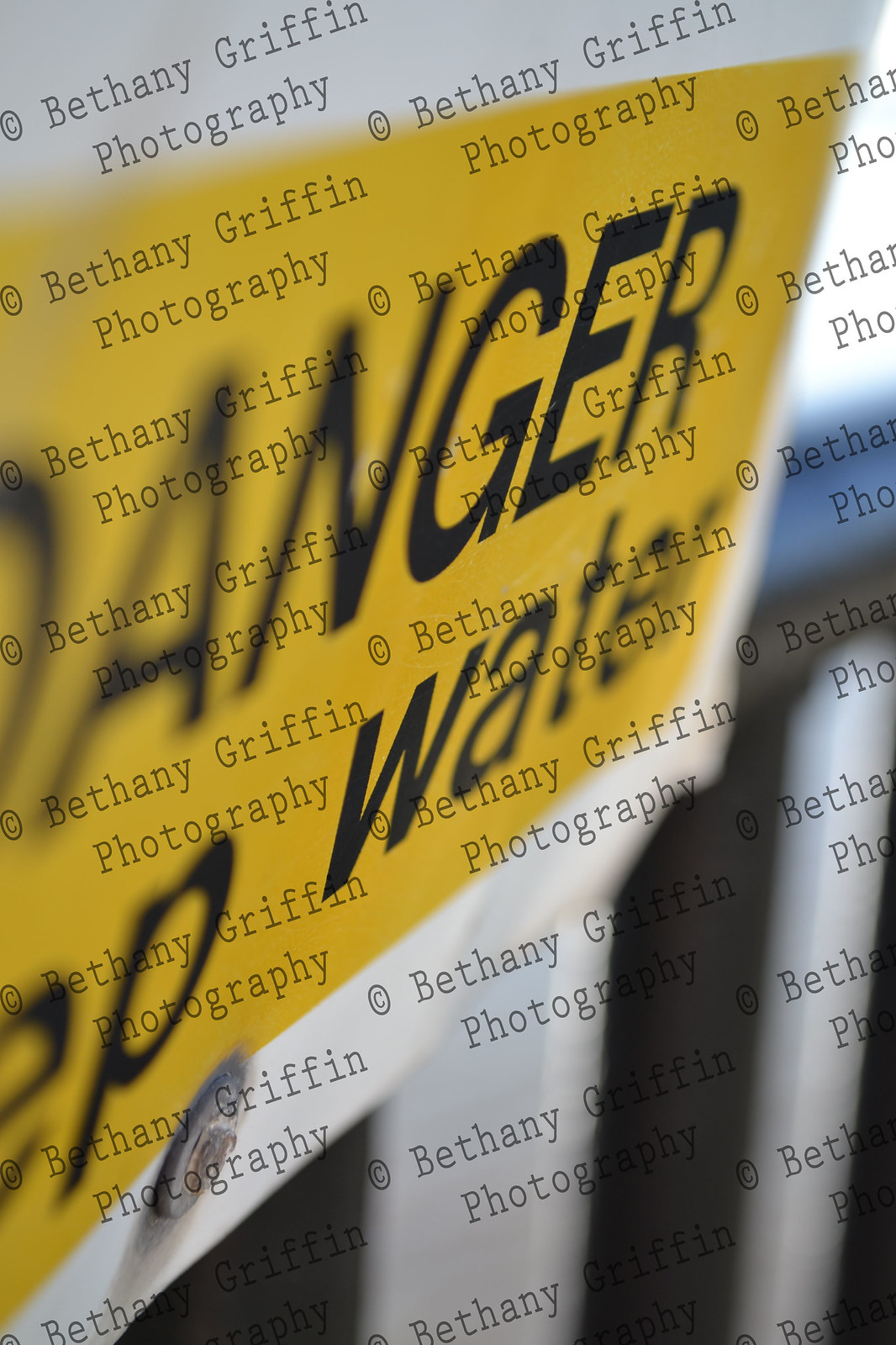The image is a close-up, collage-style graphic prominently featuring a sign that reads "Danger, Deep Water," though the "Deep" is partially obscured, showing only the "E" and "P." The word "Danger" is in black text against a yellow background, which transitions through shades of white and gray. The focus is on portions of the letters "GE" from "Danger" and "W" from "Water," while the rest of the sign appears blurry. This sign with bold black lettering is set diagonally across the image, possibly positioned next to a body of water, ground, and sky.

The overall composition includes a repetitive, diagonal watermark reading "copyright Bethany Griffin photography" in a typewritten font, covering the entire image. The watermark also extends over what resembles a white handle of the sign. The yellow block of the sign and its surrounding elements create a layered effect, suggesting the image might be an experimental overlay or collage by Bethany Griffin. The prominent watermarks and composite nature of the image strongly indicate the author's intent to emphasize copyright protection for her work.